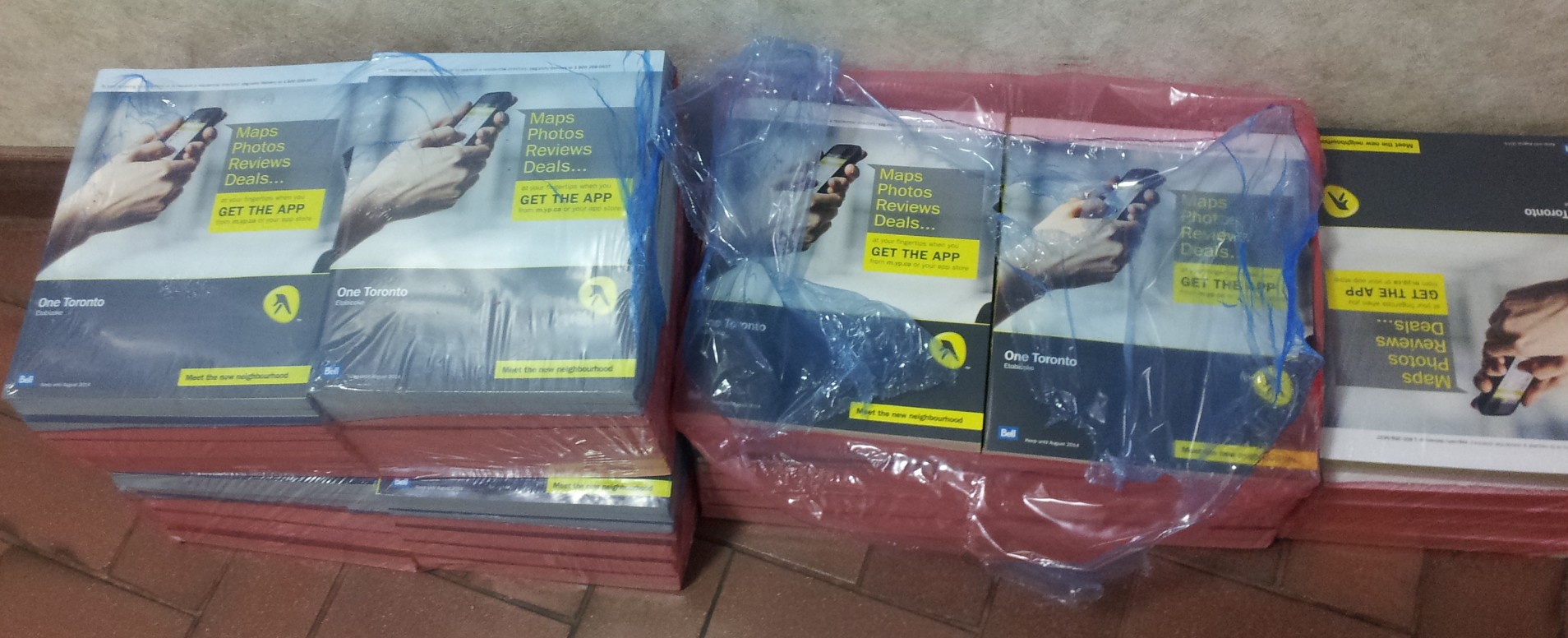The colour photograph captures several stacks of packaged books or directories, potentially phone books, arranged on a brick-red floor. There are five distinct piles, each wrapped in plastic with approximately 12 items per stack. Most of the books feature a blue cover adorned with a white image on the left, resembling an arm or hand holding a phone with a visible keypad, and a square photo on the right. The cover includes yellow text stating "Maps, Photos, Reviews, and Deals," with a bolder yellow line below reading "Get the App." The books have grey tops, and the sides appear red from below. Notably, the stack on the far right differs with a black bottom and grey top, and is upside down. Behind the stacks is a greyish, mottled wall, possibly wallpapered. The far-left and central stacks show unopened packages, while the rightmost stack appears to have some books with the plastic removed, and the top book of this stack oriented away from the viewer.